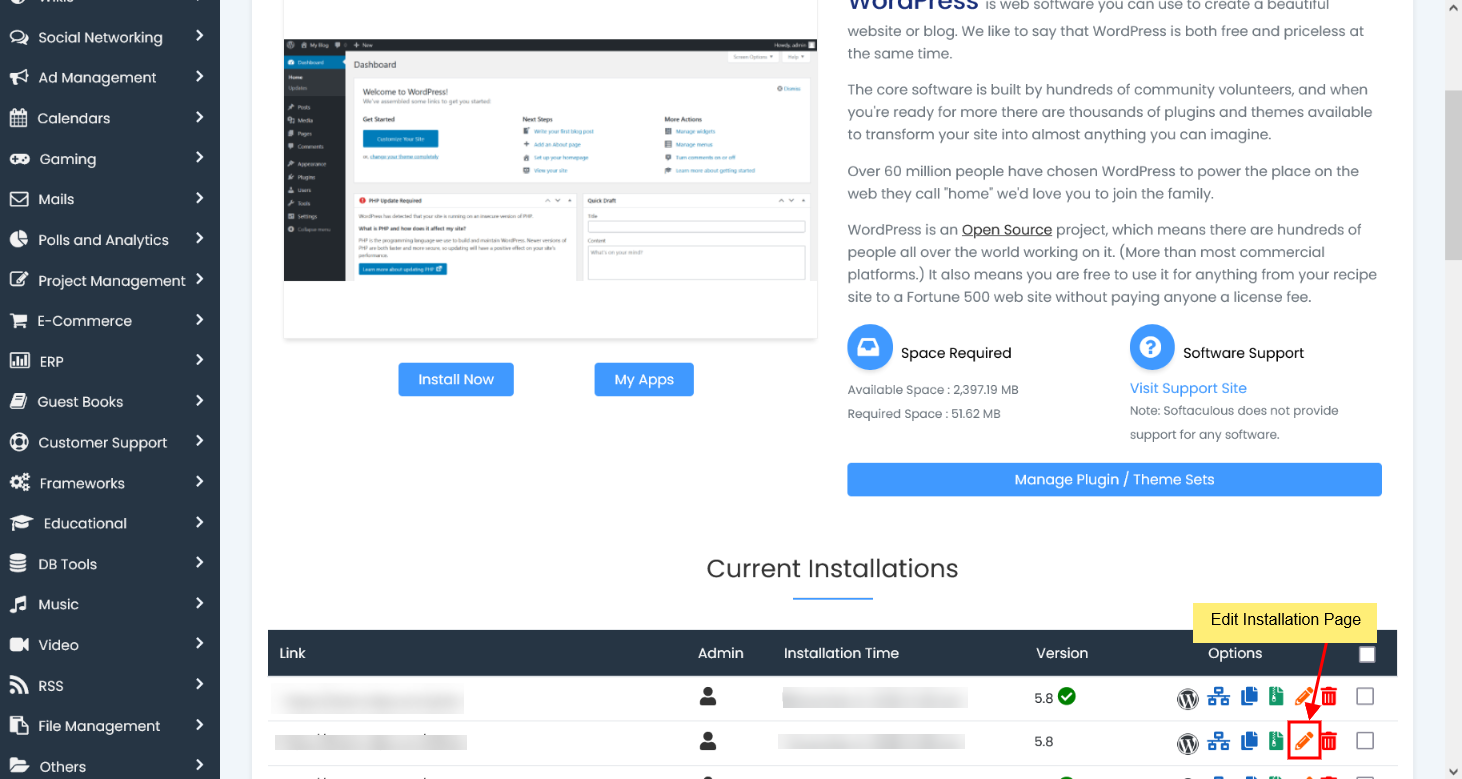The image depicts a cluttered and visually challenging user interface of an app or software with very small text and some text being cut off. The left side features a menu with a dark gray background and white text. The menu comprises the following sections, each accompanied by an illustrative icon: Social Networking, Ad Management, Calendars, Gaming, Mails, Polls and Analytics, Project Management, E-Commerce, ERP, Guest Books, Customer Support, Frameworks, Educational, DB Tools, Music, Video, RSS, and File Management. Despite the difficulty in seeing the rest of the screen clearly, it appears that this interface is associated with WordPress, suggesting that the page allows for the installation and management of WordPress on a computer.